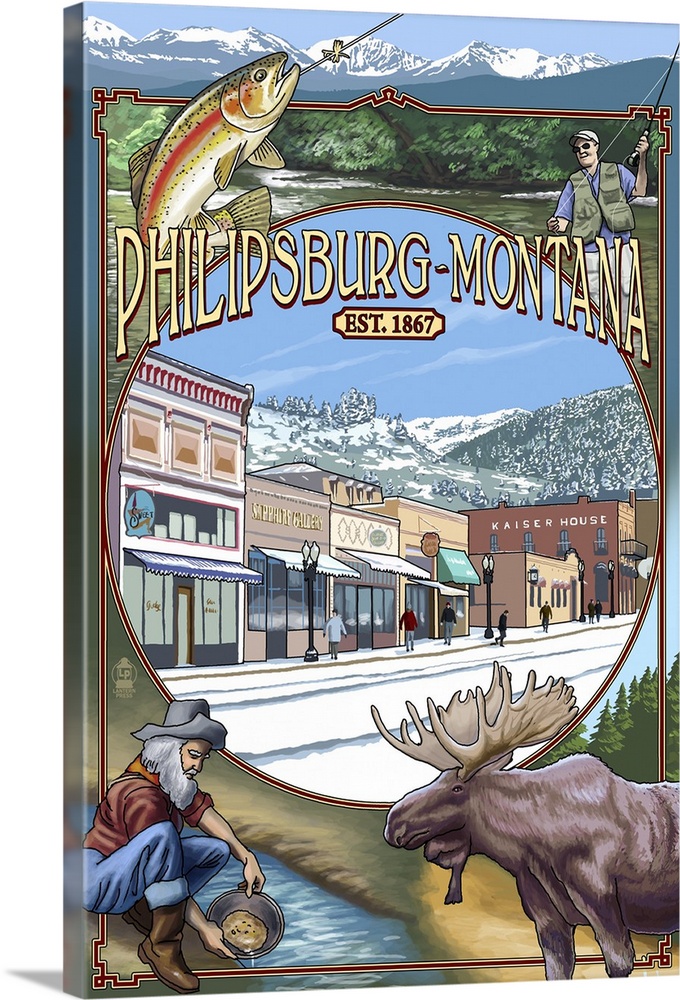The image, which appears to be the cover of a thick book styled in an Art Nouveau manner, showcases a detailed and vibrant scene dedicated to Phillipsburg, Montana, established in 1867. The top portion of the cover prominently features snow-capped mountains that cast a white hue over the landscape. Below this snowy vista, a thin red border frames the central artwork, which includes a variety of colorful, animated elements.

On the top left, a fish, possibly a trout or bass, is depicted leaping out of the water, attached to a hook whose line extends from the top center of the image, arching over the mountains. In the top right corner, a man dressed in fishing gear and wearing sunglasses is shown holding a fishing rod, which curves towards the top right edge.

Dominating the center within an oval, nearly circular frame, is a detailed illustration of a small town during winter, with rows of boxy buildings lining snow-covered streets. Above this oval frame, in large letters, is the inscription "Philipsburg-Montana," and directly beneath it, in a smaller box, "EST. 1867" is noted.

In the bottom left corner, an elderly prospector with a gray hat and white beard is depicted panning for gold in a shallow creek. Oppositely, in the bottom right corner, a majestically antlered moose faces leftward, with its body extending slightly off the right edge of the cover.

Overall, the cover's rich details and humorous Art Nouveau style pay homage to the heritage and scenic beauty of Phillipsburg, Montana.